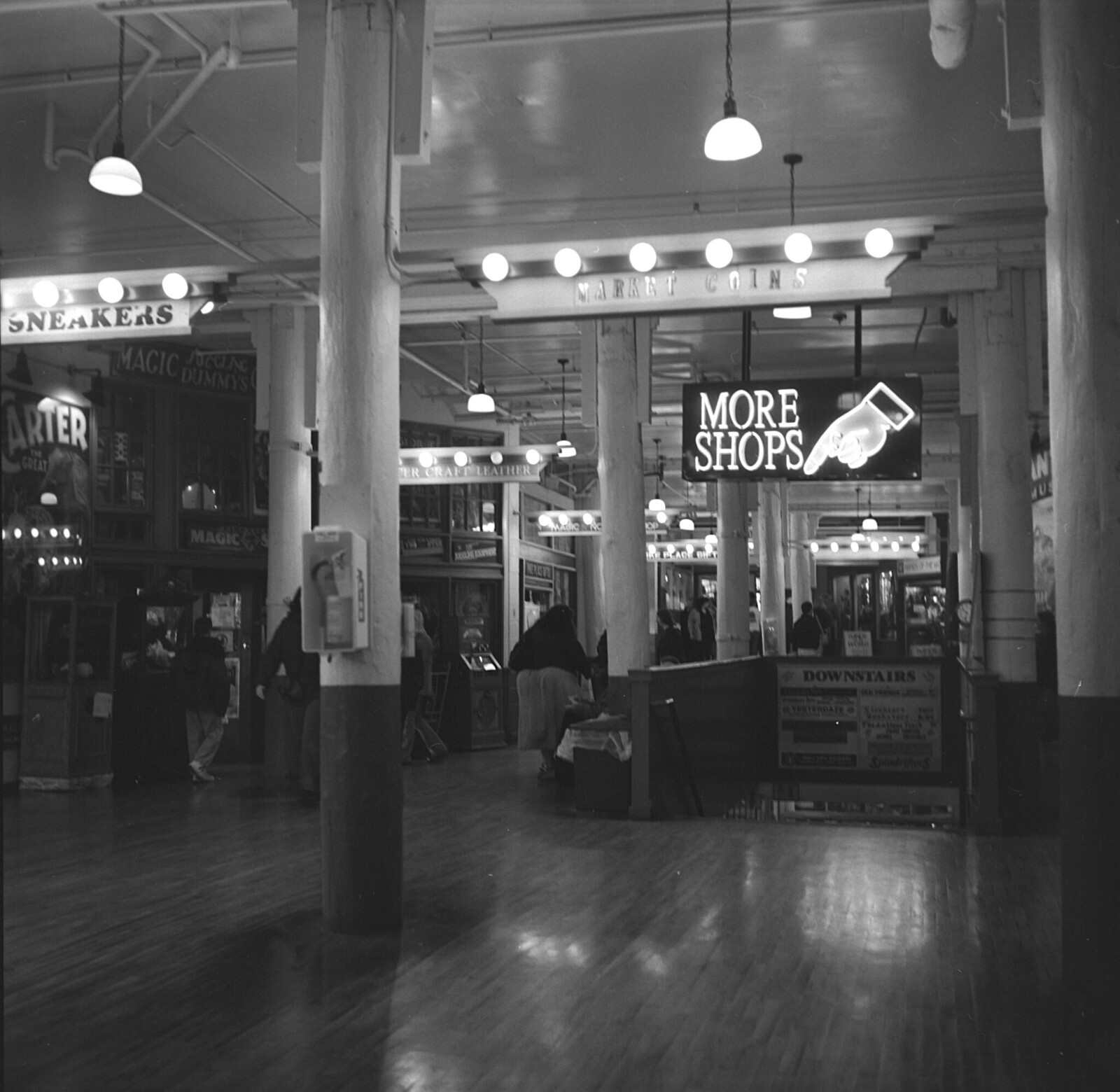This black-and-white photograph depicts the intricate exterior and inviting entrance of an early indoor marketplace, possibly reminisce of early malls. Dominated by a hardwood floor, the scene showcases a bustling sidewalk lined with various storefronts. A prominent feature is a brightly lit neon sign adorned with a pointing hand, directing visitors downstairs to "More Shops." The elegant handwriting of "More Shops" contrasts against the backdrop of round bulbs that neatly frame the building, adding a vintage charm.

The left side of the image features a sign reading "Sneakers," while other signs, such as "Craft Leather" and "Market Coins," hint at the diverse range of stores housed within the marketplace. Sturdy poles and hanging lamps add structural and aesthetic elements to the scene. In the background, beyond the illuminated signage and shop fronts, people can be seen strolling along the sidewalk, intensifying the lively and inviting atmosphere of this unique shopping center. The mixture of wooden floors, intricate signage, and bustling pedestrians encapsulates a lively and nostalgic shopping experience.